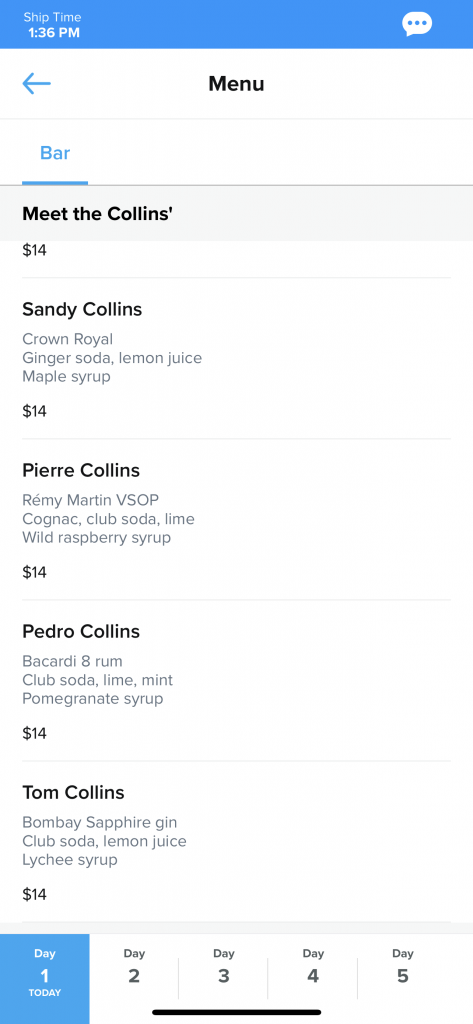The image features a menu from a bar named "Meet the Collins," showcasing a list of specialty Collins cocktails. Each drink is priced at $14 and offers a unique twist on the classic Collins recipe:

1. **Sandy Collins**: A refreshing blend of Crown Royal, ginger soda, lemon juice, and maple syrup.
2. **Pierre Collins**: A sophisticated mix of Remy Martin VSOP Cognac, club soda, lime, and wild raspberry syrup.
3. **Pedro Collins**: A vibrant concoction featuring Bacardi 8 Rum, club soda, lime, mint, and pomegranate syrup.
4. **Tom Collins**: A classic favorite composed of Bombay Sapphire Gin, club soda, lemon juice, and lychee syrup.

The menu is prominently displayed under the heading "Meet the Collins," and the "Bar" category is highlighted in blue at the center of the screen. At the bottom of the image, there is a notation indicating day numbers (1, 2, 3, 4, etc.), suggesting the menu's availability for the current day.